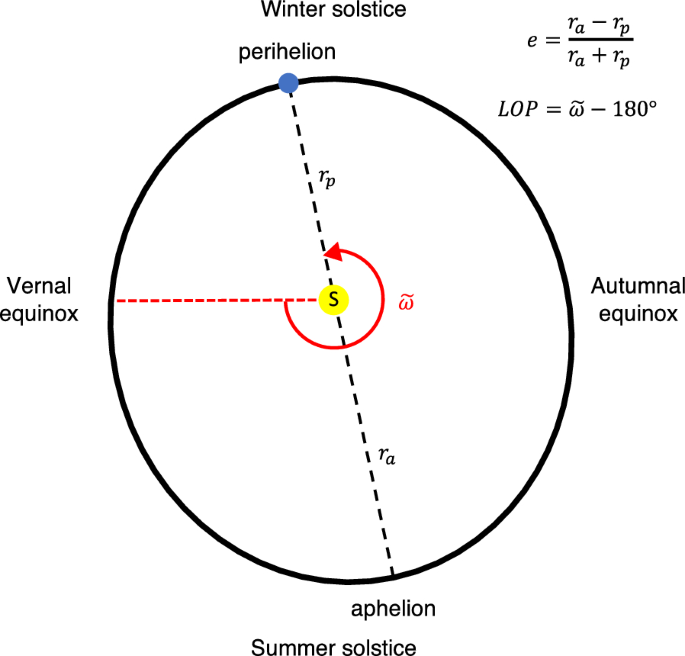This detailed diagram illustrates the celestial mechanics of the seasons, focusing on the winter solstice, summer solstice, vernal equinox, and autumnal equinox. It features a circular configuration representing the Earth's orbit. At the top of the circle is the winter solstice, marked with the perihelion directly below it. The summer solstice is positioned at the bottom, accompanied by the aphelion above it. Moving clockwise, the autumnal equinox is on the right, while the vernal equinox is on the left.

A dotted line bisects the circle vertically from the winter to the summer solstice, marked as RP (perihelion) at the top and RA (aphelion) at the bottom. A red dotted line from the vernal equinox intersects this vertical line at the circle's center, where a golden circle labeled 'S' signifies the Sun.

The diagram also includes mathematical equations in the top right corner: \( E = \frac{rA - rP}{rA + rP} \) and \( LOP = W - 180° \). These equations highlight key orbital parameters but are not explicitly detailed in their applications.

This intricate depiction of the Earth's seasonal cycle visually links the important celestial events with precise mathematical expressions and spatial relationships within the orbit.